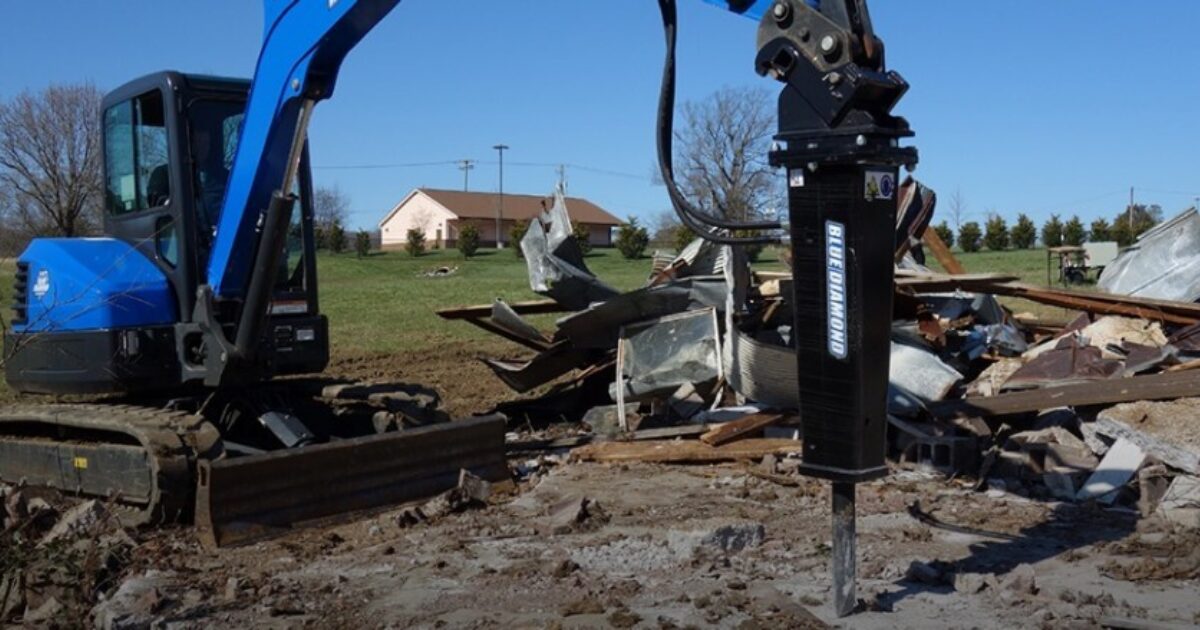The photograph depicts a daytime outdoor construction site beneath a clear blue sky. Central to the image is a compact blue and black construction vehicle, resembling a small bulldozer with a boom arm equipped with a large black drill, labeled "Blue Diamond." The drill appears to be actively breaking up concrete or hard ground in an area with evident signs of previous building demotion, such as scattered rubble including metal supports, window panes, and bricks. Surrounding the primary construction activity, there's a mix of brown dirt and green grass, with piles of debris visible to the right of the machine. In the background, a white house with a pale brown roof stands out, flanked by various green bushes and trees. Electrical poles and wires stretch across the landscape, further emphasizing the outdoor setting. Additionally, large, leafless trees are visible on the left-hand side, contrasting with the smaller bushes on the right. The overall scene combines elements of construction, demolition, and a natural environment, reflecting a busy and complex working area.